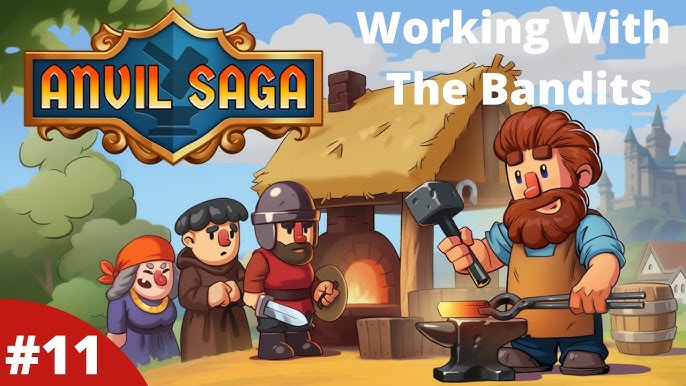The image is a detailed cartoon illustration set against a blue sky dotted with white clouds. To the left, there's a green tree, and dominating the right side, white text reads "Working with the Bandits." An emblem-like sign featuring a hammer and anvil in gold occupies the upper left corner, and in orange and yellow letters beneath it, the text "Anvil Saga" is displayed. A rounded red box with the number 11 in white is positioned in the lower left corner.

In the foreground, a muscular blacksmith, distinguished by his brownish, thick beard and hair, is in the middle of his work. His squarish facial features are notable, with a cube-like face and rectangular eyebrows. Dressed in a brown apron, a blue long-sleeved shirt with rolled-up sleeves, and blue pants paired with brown shoes, the blacksmith holds a steel hammer in his right hand and a pair of metal tongs in his left. The tongs grip a glowing yellow and reddish piece of metal, which he hammers on a steel anvil with noticeable chips on its front.

Observing the blacksmith are three medieval-looking characters to his left. Closest to him is a bearded guard clad in a red vest, gray helmet, and brown pants, holding a steel sword and a shield. Behind the guard stands a friar in a classic brown robe with visible hands held together in front of him. Completing the trio is a character in a blue-purple dress and orange handkerchief tied around her gray hair, wearing a gold necklace and sporting a big red nose—appearing somewhat pirate-like.

The background is rich with details: a straw-roofed hut with a chimney emitting smoke, a rounded fireplace with visible flames, several houses, and a distant castle to the right. The ground is yellow, contrasting with the vibrant scene, encapsulating a vividly busy medieval workshop.